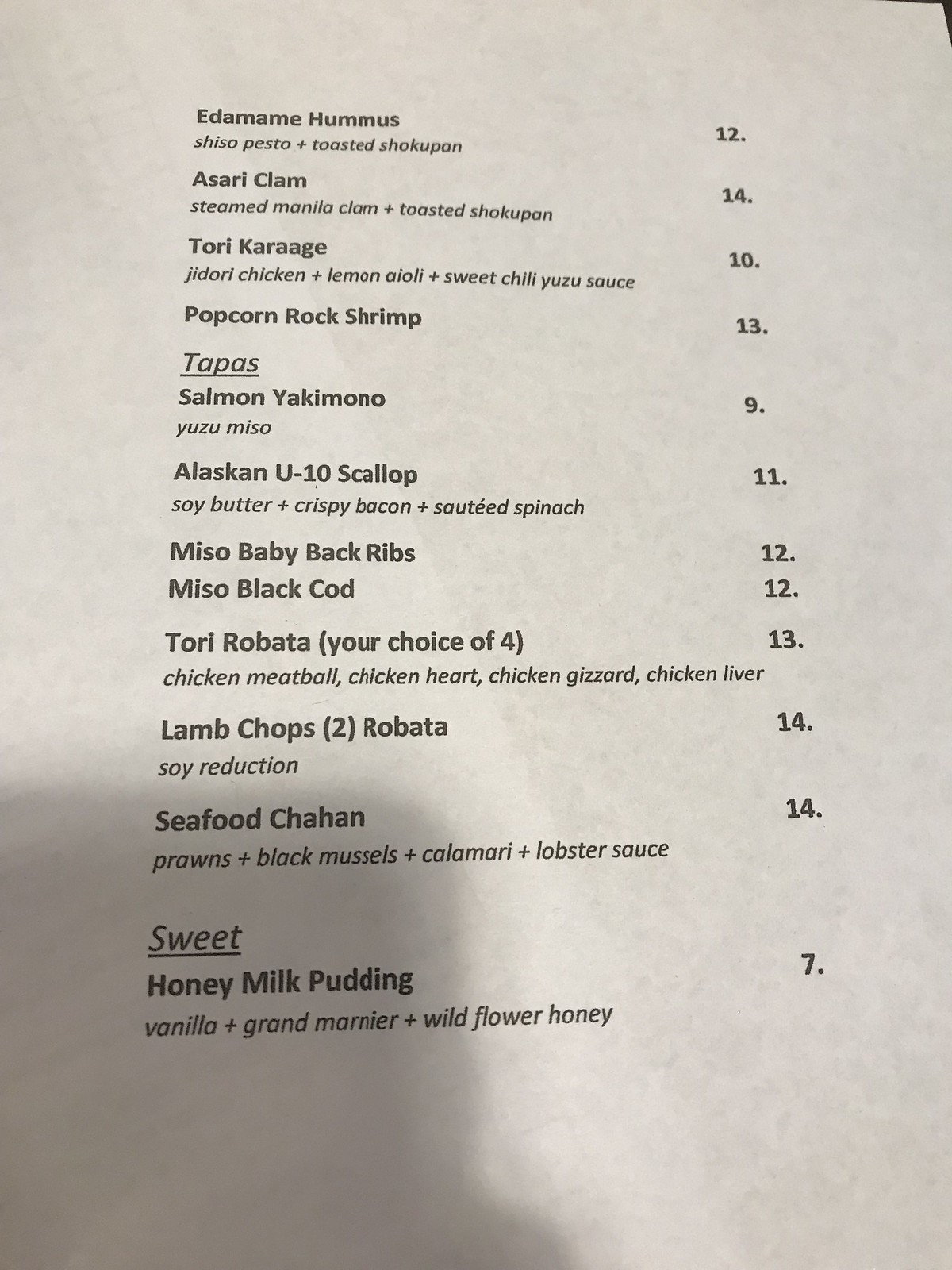This photograph captures a downward-angled view of a restaurant menu printed on white paper. In the bottom left corner, the shadow of an iPhone used to take the picture is visible, along with a faint shadow of a finger. The top right corner of the image reveals a small portion of a black background. The menu lists a variety of dishes, starting with edamame hummus priced at $12, followed by asari clam for $14, curry karaage for $10, and popcorn rock shrimp for $13. 

Under the "Tapas" section, the menu features salmon yakumo for $9, Alaskan U-10 scallop for $11, miso baby back ribs for $12, and miso black cod for $12. A selection of tori robata offers choices like chicken meatball, chicken heart, chicken gizzard, or chicken liver, each costing $4, or $13 for a combination. Lamb chops with soy reduction are priced at $14. The seafood shahan, consisting of prawns, black mussels, calamari, and lobster sauce, is available for $14. 

Finally, the "Sweets" section includes a honey milk pudding for $7.